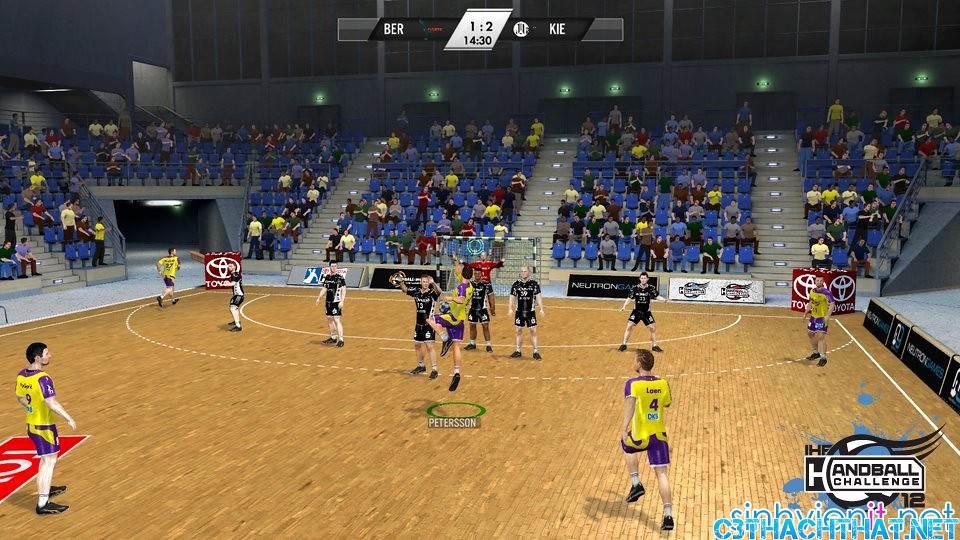The image depicts an intense handball game captured in a video game titled "Handball Challenge," as indicated in the bottom right corner of the screen. The game environment features a wooden indoor court surrounded by risers with blue seats filled with enthusiastic audience members. The players are engaged in the game, with one team clad in yellow and purple uniforms while the opposing team wears black. A red-uniformed goalie stands alert with hands raised in front of the goal net, ready to defend against any incoming shots. Prominent logos, including the Toyota logo against a red background and a pair of white cubes, are visible around the court. The in-game scoreboard at the top shows the competing teams as BER and KIE, with BER leading by 2-1 at the 14:30 mark of play. Additionally, a web URL, "C3FastChitChat.net," is noticeable in the scene.